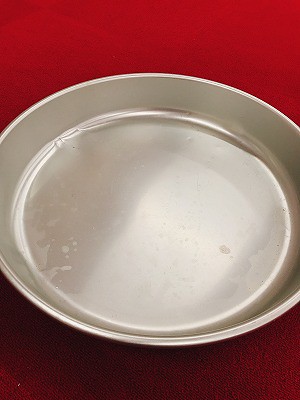This small vertical rectangular image showcases a shiny silver pie pan placed against a red background. The red hues transition from a brighter shade at the top to a dark brownish-red at the bottom. Light illuminates the pie pan more on the right side, creating a contrast with the slightly darker left side and edges. The pie pan, slightly bent along the rim, displays minor spots indicative of previous use. The red background, resembling a tablecloth, envelops the scene, emphasizing the metallic sheen and imperfections of the pie pan. The photo doesn't capture the entire pan, as its edges extend beyond the frame.